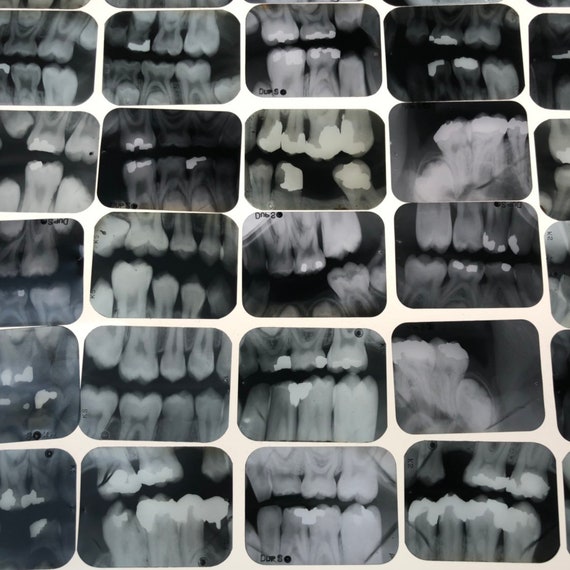This image is a detailed collage of dental x-rays, displayed in four rows with part of a row visible on the right side. The x-rays are black and white, each capturing about eight teeth in small, rectangular frames with rounded corners. They appear randomly placed on an illuminated white background, some slightly touching. The condition of the teeth varies dramatically: some x-rays show teeth in excellent shape with no visible issues, while others reveal significant problems. Highlighted white areas indicate potential cavities or plaque buildup. Several x-rays display missing or decayed teeth, and some teeth are almost hollow or require extractions. Crooked teeth and spatial issues, such as overlapping and a sideways wisdom tooth, are also evident. This assortment reflects a range of dental health conditions and stages.